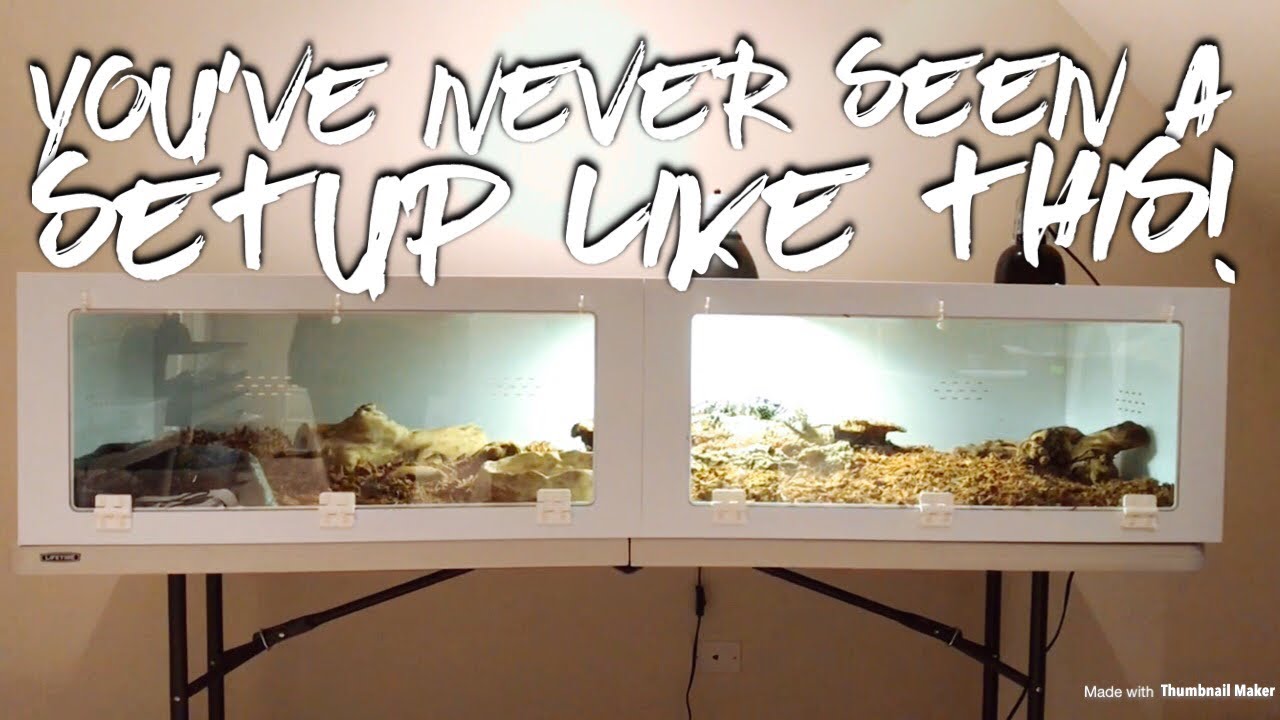The image showcases an indoor scene with beige walls and a white table with black legs positioned against the wall. The focal point of the picture is a large, elaborate reptile enclosure, mistaken by some as a fish tank, which spans the width of the table. The enclosure has a white exterior with a glass front, and inside it features typical reptile habitat elements such as substrate, rocks, and a glowing heat lamp situated in the middle. The enclosure is cleverly designed with a white slat in the center, giving the illusion of it being two separate units, but it is, in fact, a single expansive unit. The image includes a bold white caption at the top that reads "You've never seen a setup like this!", indicating that the picture was created using a thumbnail maker, possibly for a YouTube video focused on reptilian habitats.